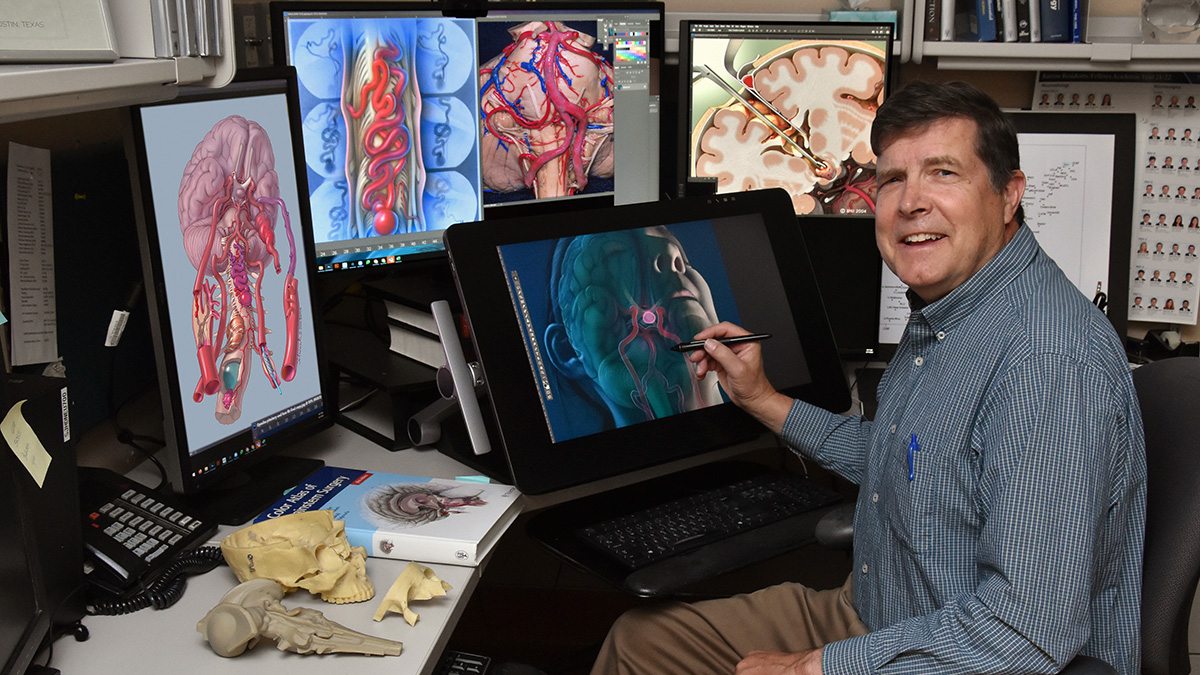This color photograph depicts a man, presumably a doctor or a digital artist, seated at his workstation. He is wearing a blue and white small-checkered button-up shirt with a blue pen clipped in the front pocket, paired with tan or brown slacks. The man, a light-skinned male with dark brown hair, is smiling at the camera, showing his teeth. 

He is engaging with a digital drawing pad using a black stylus in his right hand, while his left hand rests on his knee. Before him is an interactive monitor tilted towards him, displaying a detailed diagram of a human head, showcasing internal features such as veins and blood flow, highlighted in pink.

The workspace is surrounded by five additional screens, each depicting various medical images focused on different parts of the human body. These images include close-ups of the brain, brain stem, blood vessels, and possibly other anatomical features. To the left of his desk are various objects, including plastic models of the skull and brain stem, a telephone with gray buttons, and a open textbook, likely a "Color Atlas of Surgery."

The background includes cream-colored shelves adorned with books and other items, contributing to the office's academic and professional atmosphere. There also appears to be a binder with a yellow sticky note and papers pinned to the wall, possibly containing phone numbers or diagrams of fellow doctors. The overall setting conveys a blend of medical precision and digital artistry, likely pointing to the man’s profession in the medical field, potentially as a neurologist or a medical illustrator.